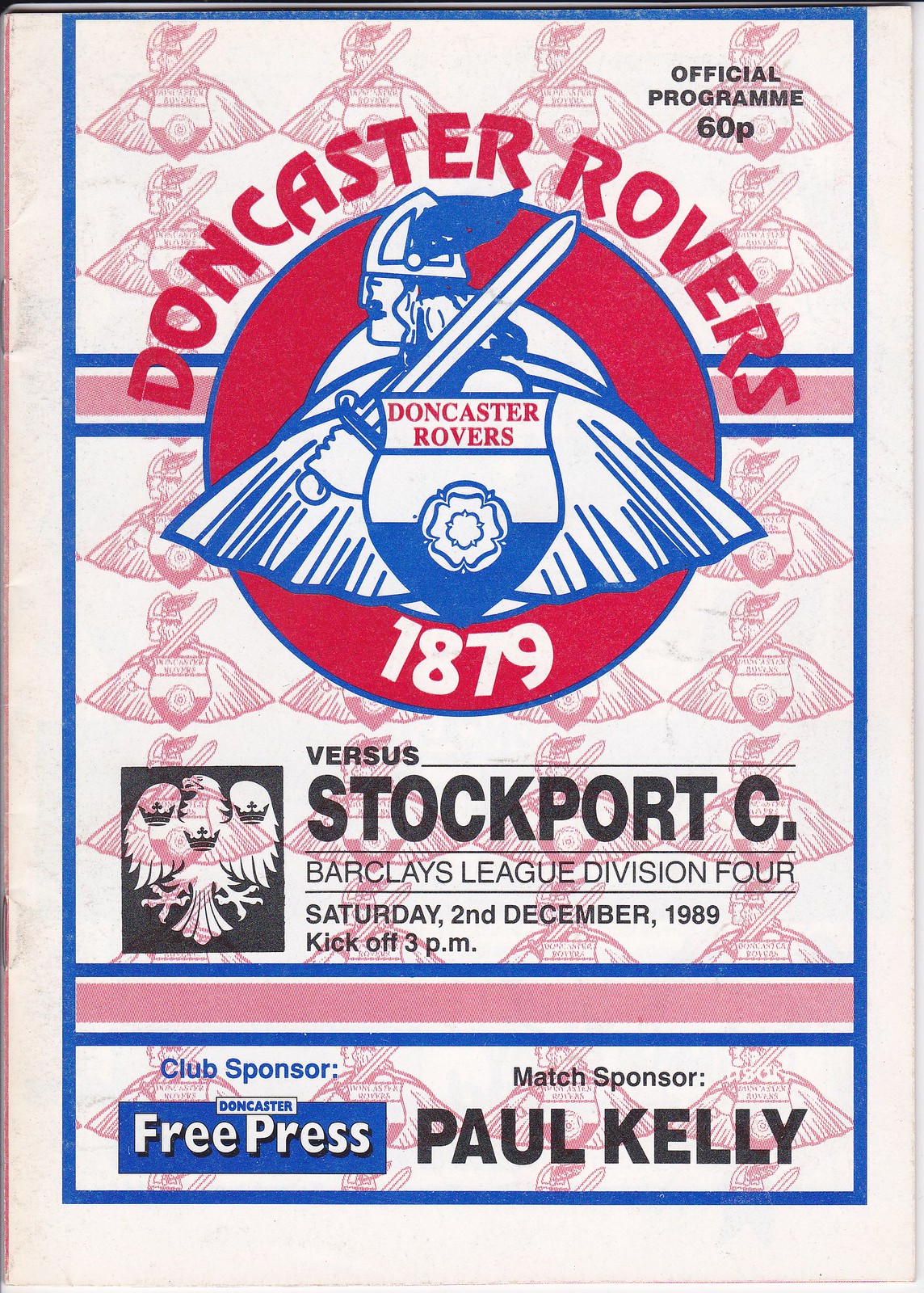This image depicts the front cover of an official matchday program for a Doncaster Rovers soccer game. The program has a blue border and appears to be stapled on the left side. At the top, "Doncaster Rovers" is written in bold red letters. Prominently featured in the middle is the team's blue logo, depicting a Viking warrior holding a sword, surrounded by a red circle. Below the logo, it states "Official Program, 60p." Additional details on the cover include the match information: "vs. Stockport C, Barclays League Division 4, Saturday, 2nd December 1989, kickoff 3pm." The upper right corner displays "Doncaster Rovers 1879." To the bottom right, it lists "Club Sponsor: Doncaster Free Press," alongside "Match Sponsor: Paul Kelly." The background of the cover has a pinkish hue, and the outer edges of the program are visible, giving a sense of the physical dimensions of the booklet.